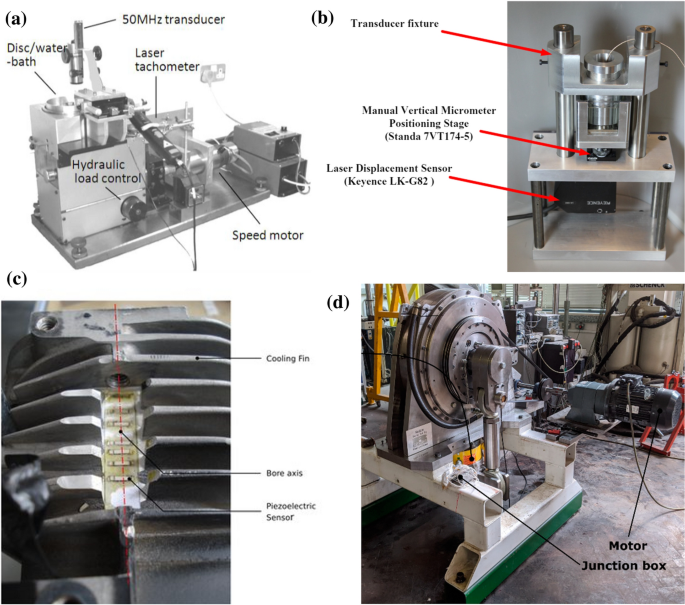This image presents a detailed quadripartite diagram of a multifaceted mechanical system, with each section labeled A, B, C, and D. 

In the top left, labeled A, a textbook-style schematic meticulously identifies various components of a structured assembly. Black text annotations highlight key parts including a 50 Megahertz transducer, a laser tachometer, a disc water bath, a speed motor, and hydraulic load control.

The top right, labeled B, provides a real-world photograph of the device. This image mirrors the schematic, with red arrows pointing to significant areas, underlined by black text labels such as a transducer fixture and a laser displacement sensor.

The bottom left, labeled C, is a close-up of a section of the apparatus resembling a metal cylinder, characterized by detailed labeling in black text for its cooling fin, bore axis, and piezoelectric sensor.

The bottom right, labeled D, shows a motor junction box situated in what appears to be a garage-like setting. Accompanying this are two large machines, one featuring a circular disk shape on a white stand labeled junction box, and another identified as a motor, supported by a red frame and indicative of classic motor design.

Through this combination of schematic and photographic representations, the image thoroughly elucidates the intricate details and configurations of the mechanical system.